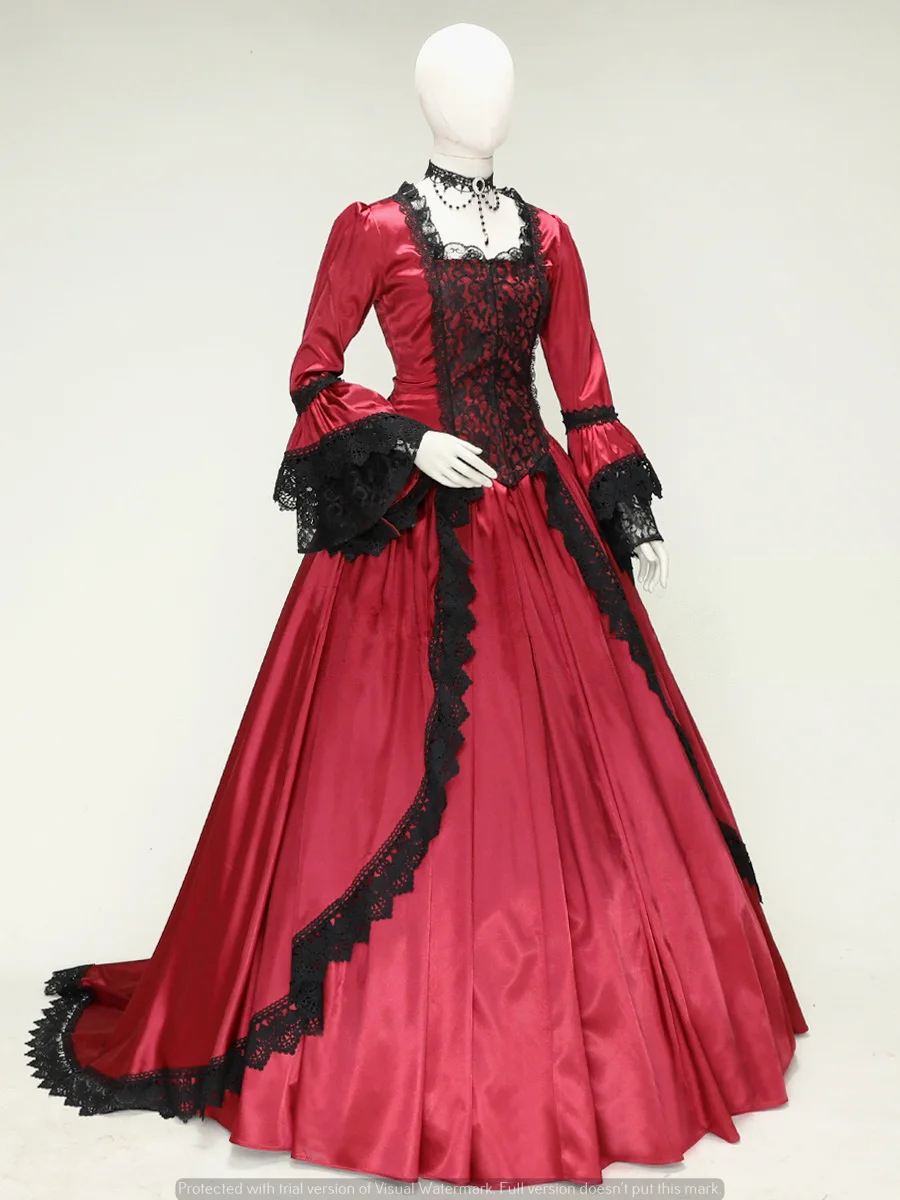This image portrays a meticulously detailed, color photograph of a formal Victorian gown displayed on a white, faceless mannequin. The mannequin, which is positioned at a slight angle toward the right, features a shiny finish and is adorned with a black lacy choker intricately designed with black beads. The gown, made of red satin, boastfully presents black lace trim throughout its design. It features a square neckline outlined by a black lace ruffle on all sides, converging onto a bodice gathered with a central black lace panel. The skirt is full-sweep, pleated, and floor-length, extending narrowly at the waist and widening at the bottom. This voluminous skirt is decorated with two overlay sections, edged in black lace, framing the central part of the skirt. The gown's sleeves start fitted and gradually bell out towards the bottom, ending in layered black lace near the hands. The background of the image is a muted greyish-beige, contributing to the gown’s visual prominence. Notably, the photograph carries a watermark with the phrase “protected with trial version of visual watermark” along the bottom, slightly detracting from the historical aesthetic of the image.